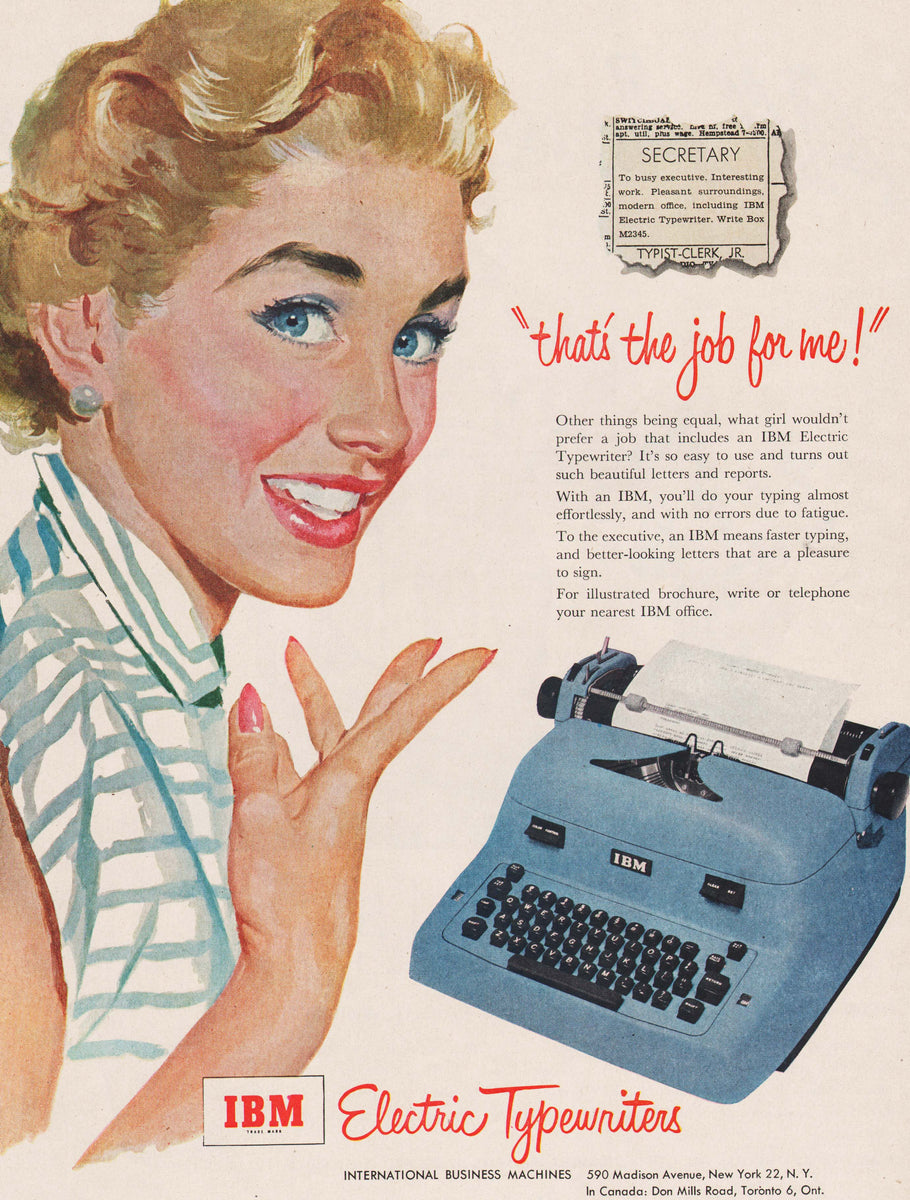This vintage watercolor-style advertisement for an IBM electric typewriter features a hand-drawn woman on the left side, reminiscent of Norman Rockwell's style and bearing a resemblance to Marilyn Monroe. She has short, wavy blonde hair, blue eyes, red lipstick, and is smiling with a joyful expression. She is wearing a teal and white striped short-sleeved shirt, with her right hand raised under her chin. 

On the right side of the vertical rectangle ad is a black emblem at the top with 'secretary' written inside. Below the emblem, red lettering in quotations states, "That's the job for me!" followed by a small paragraph of text in black writing. At the bottom right corner, there is an illustration of an old IBM typewriter, blue in color with black keys and a piece of paper inserted. In the bottom center of the ad, a red rectangular box contains the IBM logo, next to which 'electric typewriter' is written in red cursive lettering, accompanied by a few lines of smaller black text.